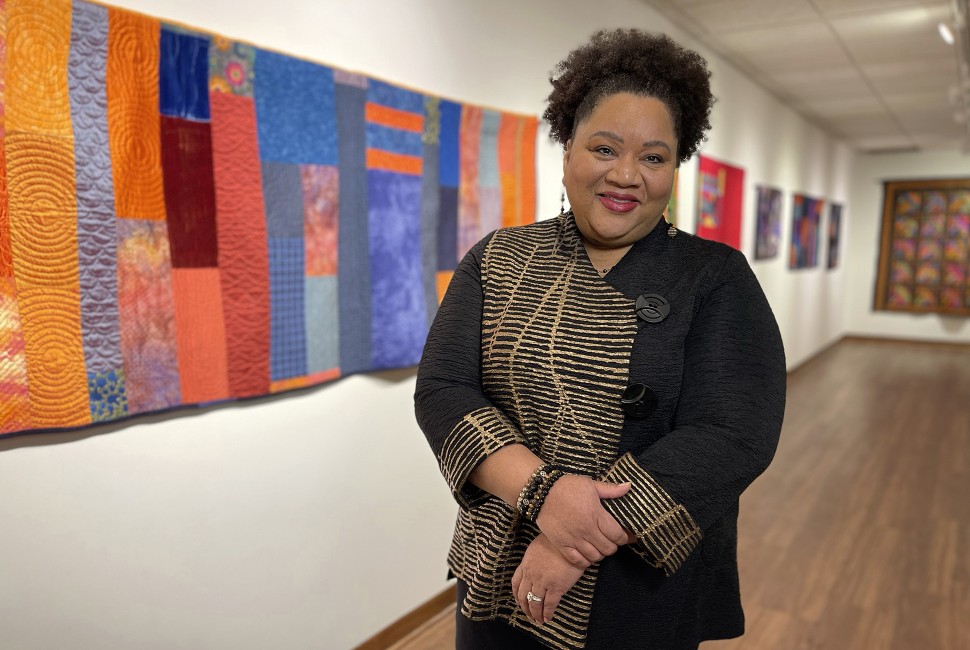In this image, we see an African-American woman standing prominently in the center of what appears to be an art gallery with white walls adorned with various colorful textiles and artworks. The textiles display a vivid array of colors, including orange, burgundy, blue, red, pink, and tangerine, all sewn together in intricate patterns. The floor beneath her is made of dark brown wood, adding warmth to the setting.

The woman is dressed in a distinctive black blouse that features light brown stripes on the body and at the ends of the sleeves. One side of her chest showcases goldish light brown swirls, complementing the solid black fabric of the rest of her top. She accessorizes with black beaded bracelets, brown and black beaded earrings, and an engagement ring on her ring finger, suggesting she is engaged or married.

Her makeup is subtle but noticeable, with her slightly open mouth revealing a hint of a smile and her lips covered in lipstick. Her black hair is styled up in a ponytail, adding to her elegant appearance.